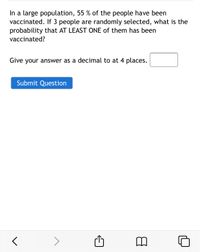The image captures a section of a web page that primarily features a white background with various interactive elements. Central to the image is a black text message conveying, "In a large population, 55% of the people have been vaccinated. If three people are randomly selected, what is the probability that at least one of them has been vaccinated? Give your answer as a decimal to at least four places." Adjacent to this text is an empty text box intended for user input. Below this, a prominent blue button labeled "Submit" invites users to answer the question. At the very bottom of the image, navigation arrows indicate options to proceed to the next page or return to the previous one.